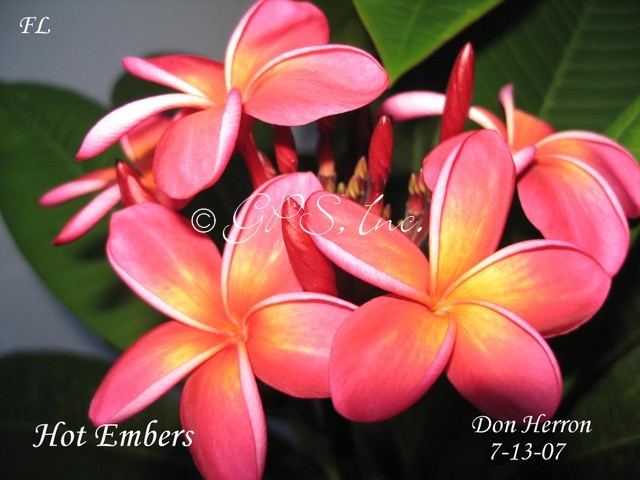The image depicts vibrant pink flowers with yellowish centers and lighter pink edges, set against a backdrop of large, lush green leaves. There are five distinct flowers, with one slightly obscured in the background. Deep red, cylindrical buds also extend upwards from the plant. The background is a muted gray, adding contrast to the bright flora. White text features prominently in three areas: the upper left corner displays "FL," the bottom left corner reads "hot embers," and the bottom right corner notes "Don Heron 71307." Additionally, a subtle watermark in the center states "copyright GPS, L&C, Inc."